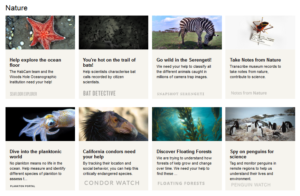**Detailed Caption:**

This screenshot captures a website interface accessed on a landscape-oriented device, likely a desktop, laptop, or tablet. The webpage focuses on the theme of "Nature," prominently featured in a heading at the top. Below this heading, the page is divided into two rows containing a total of eight images, each showcasing different animals, sea creatures, or insects, accompanied by brief descriptions.

In the first row, from left to right:
1. A clear photograph of a starfish with the caption "Help Explore the Ocean Floor," followed by additional unreadable text.
2. A dark, indistinguishable image with unreadable words.
3. A zebra with its head lowered, seemingly grazing on grass, with an inscription that appears to say "Go Wild in the Serengeti."
4. An image of an unidentified insect, with unreadable accompanying text.

In the second row, from left to right:
1. An unclear sea creature with unreadable words beneath it.
2. A primate, possibly an orangutan, again with unreadable text beneath it.
3. A scene from underwater with text that seems to suggest "Discover Floating Something," though the exact words are indistinct.
4. A photograph that likely depicts penguins, with unreadable words below the image.

The website design is heavily image-centered, intended to draw attention to the natural world, although the small text is largely illegible in the screenshot.